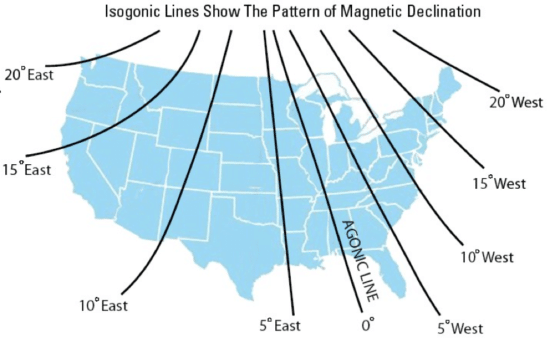The image depicts a rectangular map of the contiguous United States in light blue with white state borders, set against a bright, clear white background. The map is overlaid with black isogonic lines indicating the pattern of magnetic declination across the country. These lines, both straight and arc-shaped, are labeled at various intervals. From left to right, the lines are marked as 20 degrees west, 15 degrees west, 10 degrees west, 5 degrees west, 0 degrees (agnic line), 5 degrees east, 10 degrees east, 15 degrees east, and 20 degrees east. The title at the top center of the image reads in black sans serif font, "Isogonic lines show the pattern of magnetic declination." The lines fan out radially from top center to various angles, with some extending towards the Gulf of Mexico and the Atlantic Ocean, creating a detailed and visually informative diagram of magnetic declination within the United States. Notably, the map only includes the 48 contiguous states, excluding Alaska and Hawaii.